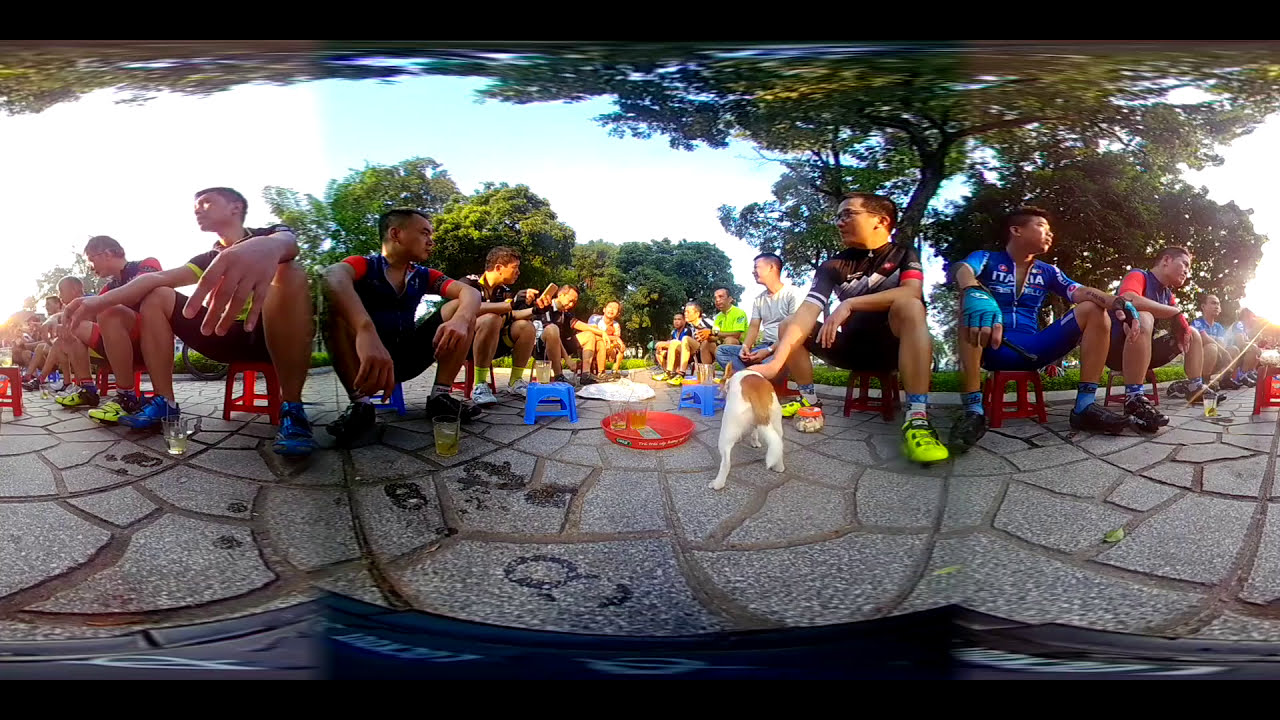The panorama image depicts a group of men dressed in professional biking outfits, seated on small red stools arranged in two groups within a public park. They are positioned on a long, paved, gray cobblestone plaza, surrounded by dense green trees under a clear, bright blue sky with some clouds. A few men appear to be holding their phones or engaging in light conversation while waiting. Notably, one man on the right is wearing an outfit that says "Italia." In the center, a small, white dog with a brown tail is being petted by one of the men, and nearby, a red bowl holds two half-full glasses. The overall scene suggests a gathering or rest stop, with the men lounging and enjoying the sunny day.